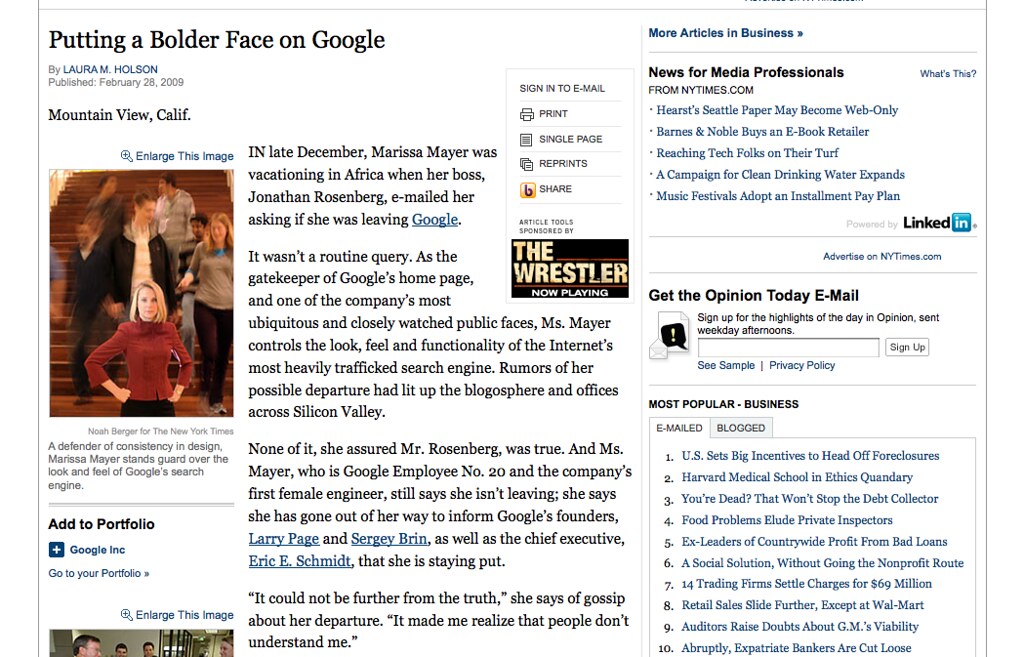**Caption:**

A screenshot from an unknown source highlights an article by Laura M. Holson titled "Putting a Bolder Face on Google," published on February 28, 2009, in Mountain View, California. The focus of the piece is Marissa Meyer, Google's first female engineer and employee number 20. While vacationing in Africa in late December, Meyer received an email from her boss, Jonathan Rosenberg, inquiring about rumors of her departure from Google. Meyer, who is instrumental in managing the look, feel, and functionality of Google’s homepage, assures that the rumors are false and emphasizes her dedication to staying with the company. She has communicated her intentions to Google’s founders and CEO, emphasizing that the gossip is far from the truth.

To the left is a photograph of Marissa Meyer, captured by Noah Berger for The New York Times. Meyer, a fair-skinned woman with blonde hair styled in a shoulder-length bob, stands confidently in front of a staircase filled with slightly blurred, descending people. Dressed in a long-sleeved red top with her fists on her hips, Meyer’s outfit is completed with what appears to be black bottoms. The caption underneath the photograph describes her as a defender of consistency in design and a guardian of Google’s search engine aesthetics.

To the right of the image, an area titled "More Articles in Business" lists additional news and updates from The New York Times. This section covers various headlines, such as Hearst’s potential transition to a subscription-only model for Seattle paper, Barnes & Noble’s acquisition of an e-book retailer, and other notable topics. It also includes promotional content for the New York Times, advertising sign-ups for daily opinion email highlights and more business-related news. A "Most Popular in Business" list features the top ten business stories, ranging from incentives to prevent foreclosures to questions about GM’s viability, providing a snapshot of critical economic issues at the time.